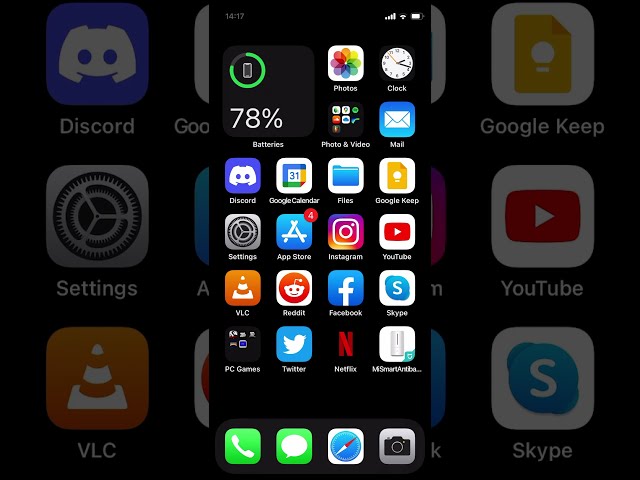A detailed caption for the image could be:

"This image features a phone screenshot prominently displayed in the center, set against an enlarged background of the same screenshot, creating a layered visual effect. The phone's battery is at 78%, and the screen showcases a diverse array of apps and utilities. Key icons include Discord, VLC, Skype, YouTube, Google Keep, Photos, Clock, Mail, Discord, Google Calendar, Files, App Store, Instagram, Reddit, Facebook, PC Games, Twitter, Netflix, and 'My Smart Anti-something,' alongside essential apps like Safari, Phone, and the green Call and Text buttons. The entire composition is presented in Dark Mode, with the black background making the colorful app icons stand out vividly. This artistic capture not only highlights various popular applications but also showcases the organizational layout of a tech-savvy user’s mobile device."